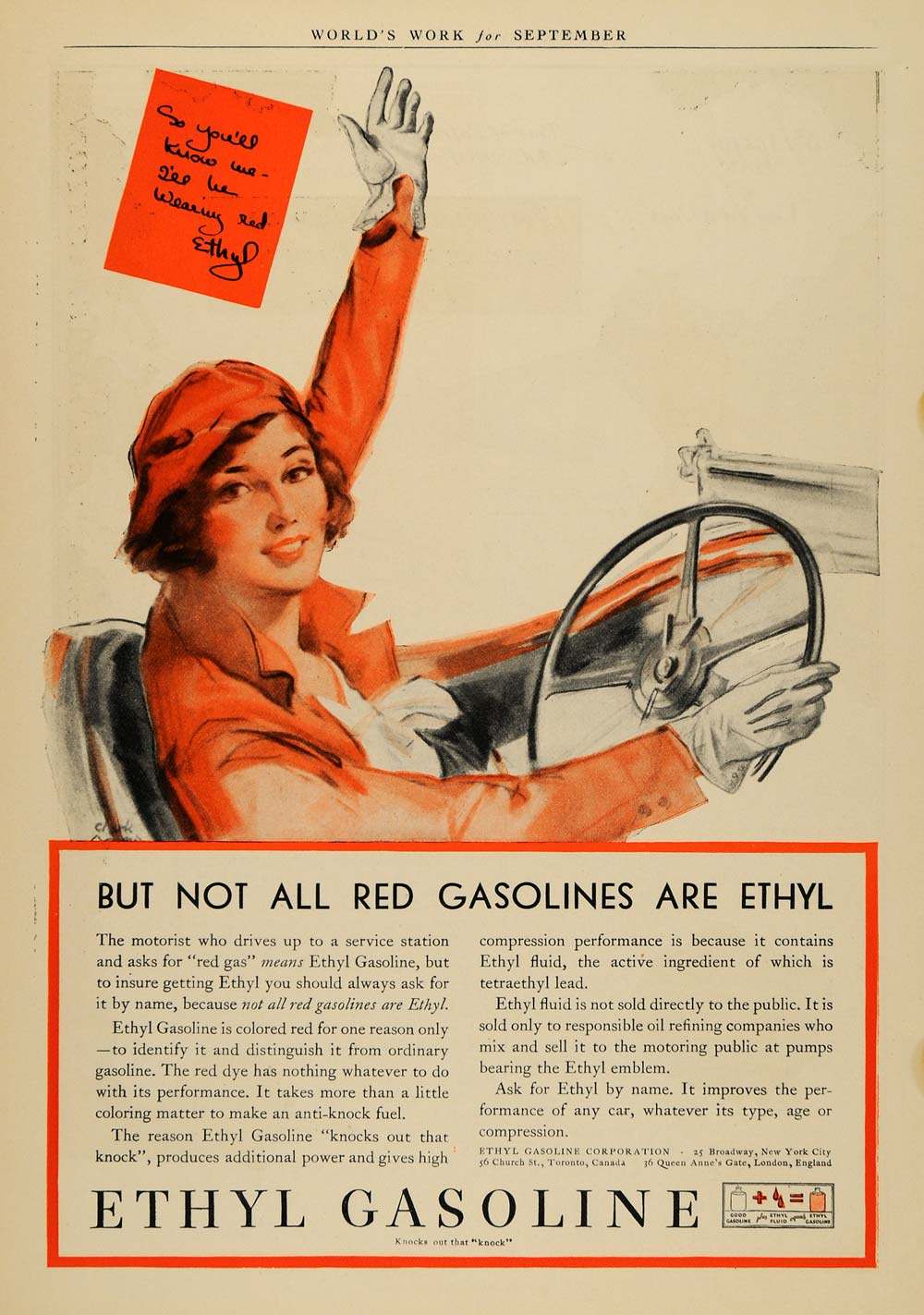This vintage magazine advertisement, likely from the 1930s or 1940s, promotes Ethyl Gasoline. The full-page ad features a detailed, painted illustration of a young woman sitting in a sporty convertible. She is depicted with a warmly smiling expression, wearing a matching reddish-orange beret and dress jacket with white gloves, and grasping the steering wheel. A prominent red note in the top section reads, "So you'll know me, I'll be wearing red, Ethyl," adding a playful, personified twist linking the woman to the gasoline brand. Additionally, the ad states "World's Work for September" at the very top. The lower section includes text explaining that not all red gasolines are genuine Ethyl Gasoline and emphasizes the importance of requesting it by name to guarantee its anti-knock performance, attributed to its content of tetraethyl lead. The advertisement underscores that Ethyl Gasoline's red color is solely for identification purposes and does not influence its efficiency.